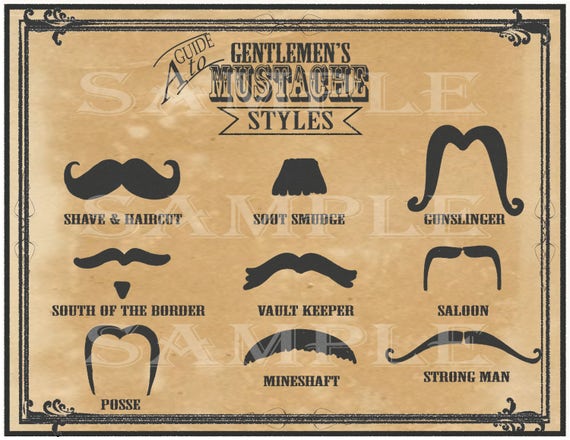This is a detailed illustration serving as a guide to various gentleman's mustache styles, rendered in black ink on a vintage, parchment-like brown background. The top of the rectangular image features the title "A Guide to Gentlemen's Mustache Styles" in an assortment of old-style fonts. The design is adorned with a double-lined border accented by scrolling flourishes in the corners. Overlaying the image are several "sample" watermarks in white/off-white, indicative of its sample status.

The guide showcases nine distinct mustache styles, each accompanied by an illustration of the mustache itself, which exhibits the bilateral symmetry characteristic of such facial hair. Arranged in three rows of three, the styles are labeled as follows: 

- Top row: Shave and Haircut, Smudge, Gunslinger
- Middle row: South of the Border, Vault Keeper, Saloon
- Bottom row: Posse, Mineshaft, Strongman

Each labeled style is meticulously detailed, providing a comprehensive visual reference for enthusiasts and aficionados of facial grooming. The entire presentation evokes a nostalgic, vintage feel through its use of parchment coloring and classic design elements.